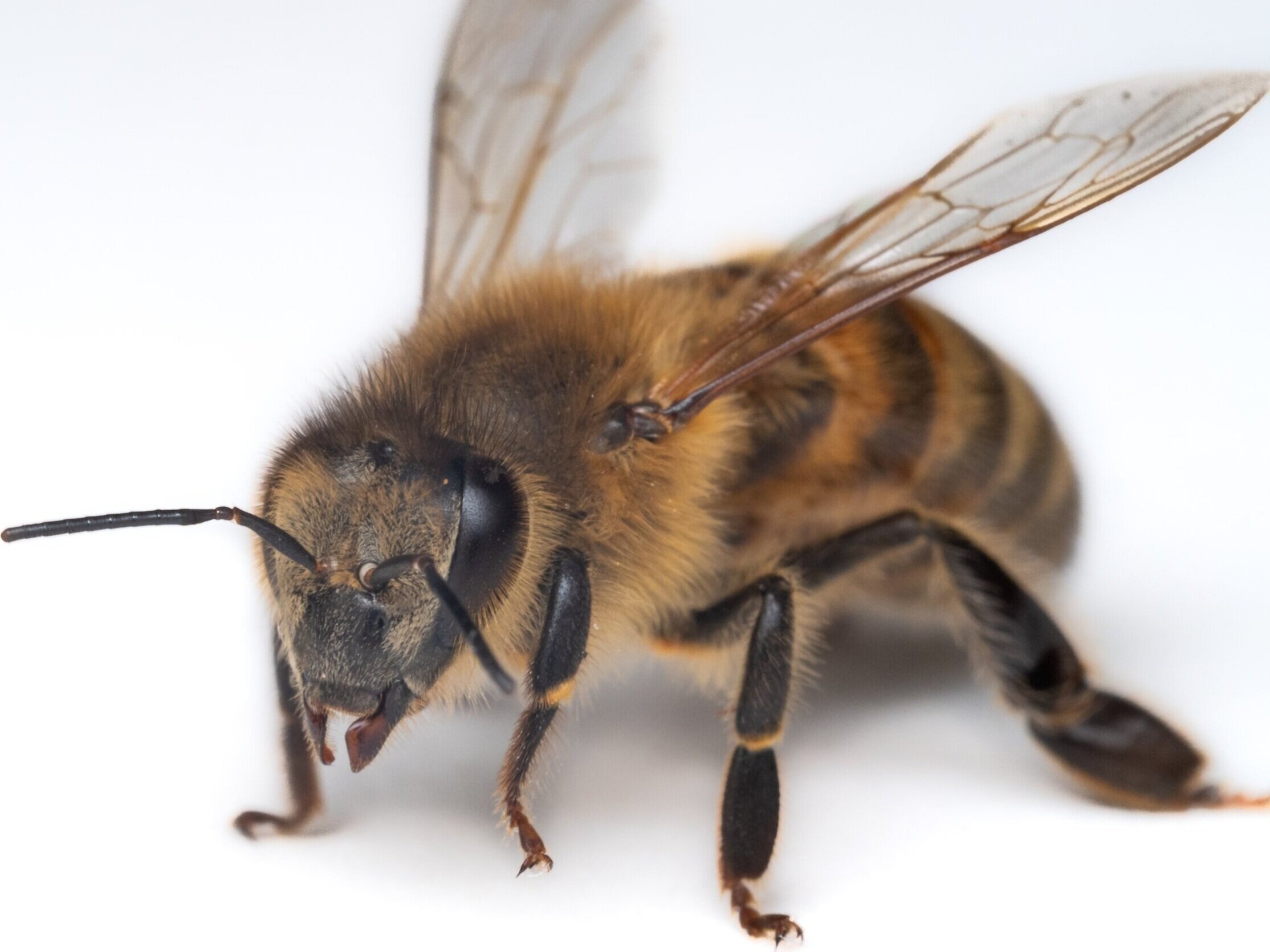This is a close-up color photograph of a honeybee captured from a front and side view against a light blue background. The bee's basic body is predominantly black with brown-colored fur covering it. Its thorax exhibits a pattern of golden and black furriness in lines, while the abdomen features interspersed light gray and golden stripes. The honeybee's antennae are jointed and black, with hints of golden at the joints, extending forward from its head. It has large black eyes and mandibles that are a mix of brown and black. The bee's legs are similarly colored with shiny black lower portions and brown, hairy upper portions. It is in a standing position, and its translucent, semi-transparent wings, held upward, show light brown veins. The wings, along with the shadow it casts on the light blue background, add to the detailed and textured appearance of this insect.